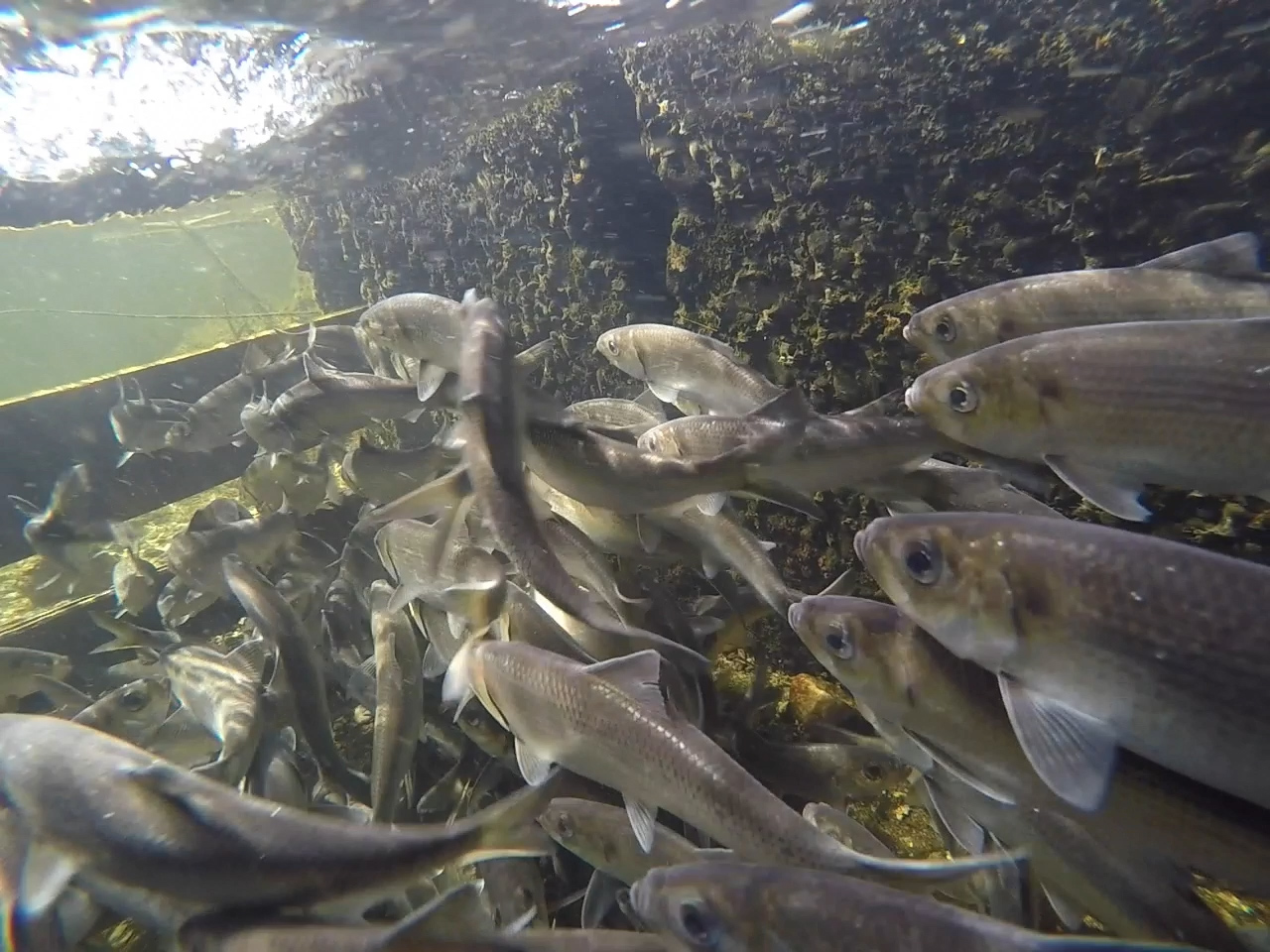The image depicts an underwater scene showcasing a large school of fish, around 20 to 30 in number, swimming rapidly in the same direction. These fish, characterized by their silvery-gray coloration, are clustered together, indicative of their natural schooling behavior. The environment appears to be shallow water, possibly an aquarium, given the presence of a partition and a rock wall on the right side. This rock serves as a backdrop, and next to it, dark green aquatic plants, resembling kelp or large weeds, add to the naturalistic setting. The image captures a dynamic moment, likely taken by someone with an interest in underwater wildlife, as the translucent partition hints at more water or a different area beyond it.